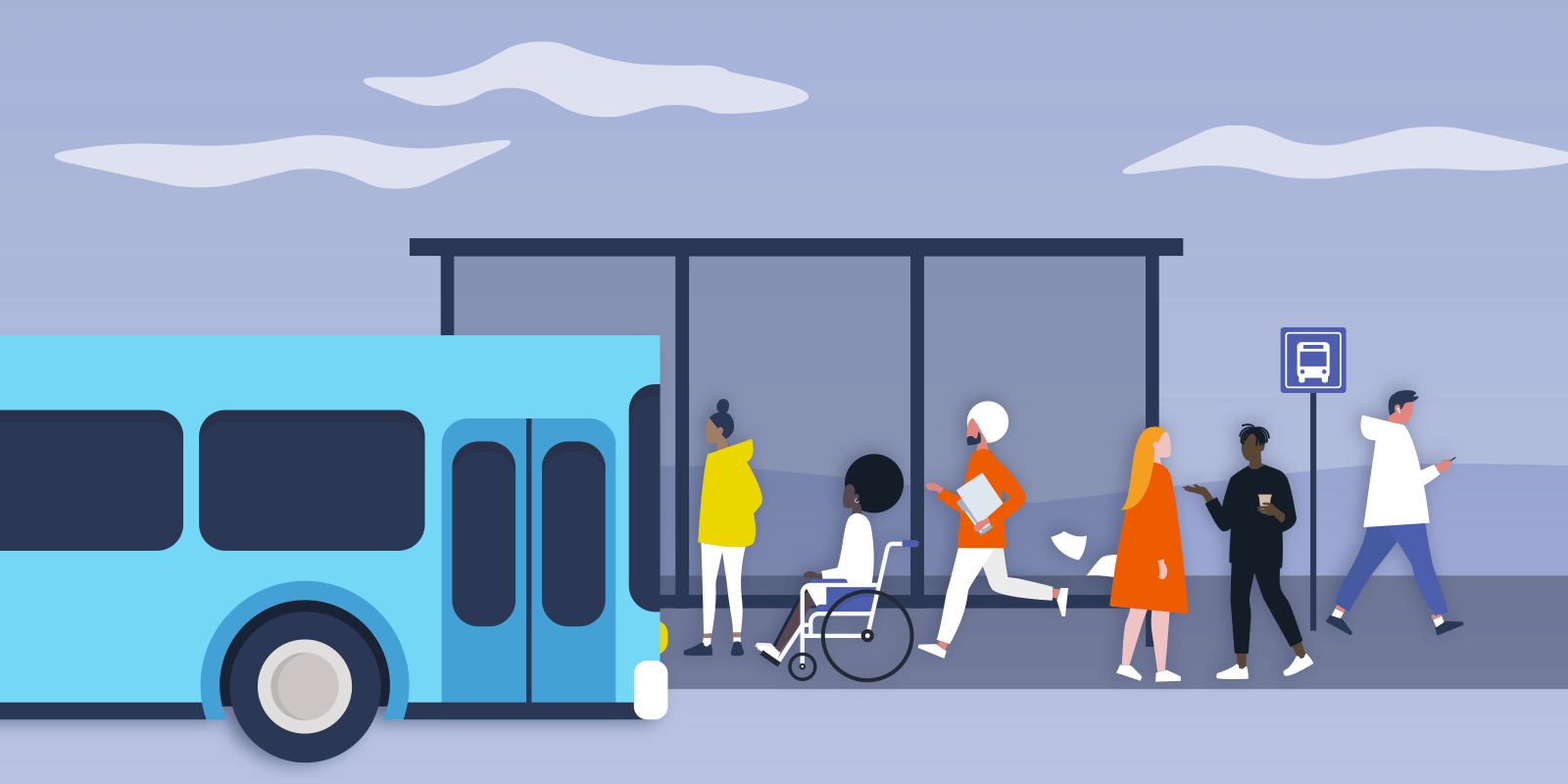The image is a rectangular graphic with a cartoon-like, cut-out paper style, depicting a bus stop scene. The light gray road contrasts with the darker gray sidewalk on which six diverse individuals are waiting. Behind them, hills with a purple-gray hue rise under a sky streaked with three wispy white clouds against a blend of blue, gray, and purple tones.

At the bus stop, a structure in navy blue shelters the characters. Approaching from the left is a partially visible turquoise bus with navy blue windows and darker blue detailing.

Among the group stands a woman in a yellow sweatshirt, white pants, and a black bun. Next to her is a black woman with a large afro, seated in a blue wheelchair with dark blue wheels. A man wearing a white turban and orange top, complemented by white pants and shoes, runs towards the bus, holding a book. A young girl in an orange coat, bare legs, white shoes, and long blonde hair is seen conversing with an afro-haired individual dressed in a navy blue sweatsuit and white shoes. Another man, donning a white hoodie, blue pants, and blue shoes with white socks, walks away from the scene, seemingly engrossed in his phone and wearing earbuds.